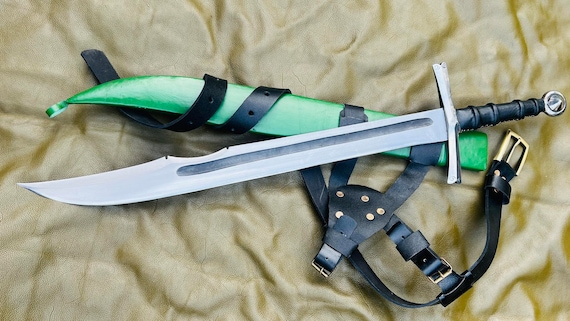This photorealistic image features a silver sword resting atop a deep green scabbard, both set diagonally on a wrinkled gold blanket. The sword has a distinct silver cross guard and a black handle adorned with four small black rings, culminating in a small silver decoration at the base of the hilt. The blade is sharp and pointed with a slight indentation near the top, running three-quarters of the way up from the handle. The green scabbard is wrapped in a black belt that extends downward to the bottom right of the image, connecting to an oval-shaped leather section decorated with five gold bolts. The gold blanket beneath shows varying shades of gold, appearing brighter in the bottom right and fading slightly towards the top left, adding depth and texture to the scene.